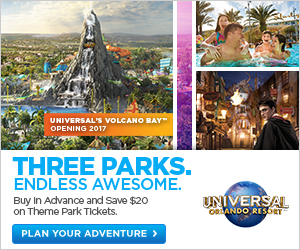This advertisement for a theme park prominently features an engaging and vibrant visual layout. The top two-thirds of the advertisement is occupied by a picturesque image, divided into three segments. The left segment features a large picture that stretches halfway across the width. A white border with a decorative pink-to-purple gradient frames this central image. The right segment is bordered by another white margin. 

At the top of the main image, a clear blue sky sets the scene. Dominating the center portion, a magnificent white mountain nearly reaches the top of the frame, crowned with a cascading waterfall. In the bottom right corner, an orange tab gradient stands out, starting from light orange and transitioning to a darker shade, featuring the text "Universal’s Volcano Bay" and the opening year "2017."

In the left top image, a joyful family—a man and woman with their kids on their back—is depicted outdoors, surrounded by two palm trees against a backdrop of the sky. Below this, another image captures Harry Potter from the back, gazing towards the camera with scenery from the movie in the background.

The bottom third of the advertisement features a clean white background with various textual elements. On the right side, bold all-caps blue letters proclaim, "THREE PARKS." Beneath this, in smaller but still prominent blue text, is the slogan "Endless Awesome." Further down in small black letters is a promotion that reads, "Buy in advance and save $20 on theme park tickets."

In the bottom left corner, a blue tab carries the message "Plan your adventure" in white letters, accompanied by a right-pointing arrow. To the right, an image of the Universal globe has the text "Universal Orlando Resort" boldly displayed across it in white letters with gold borders.